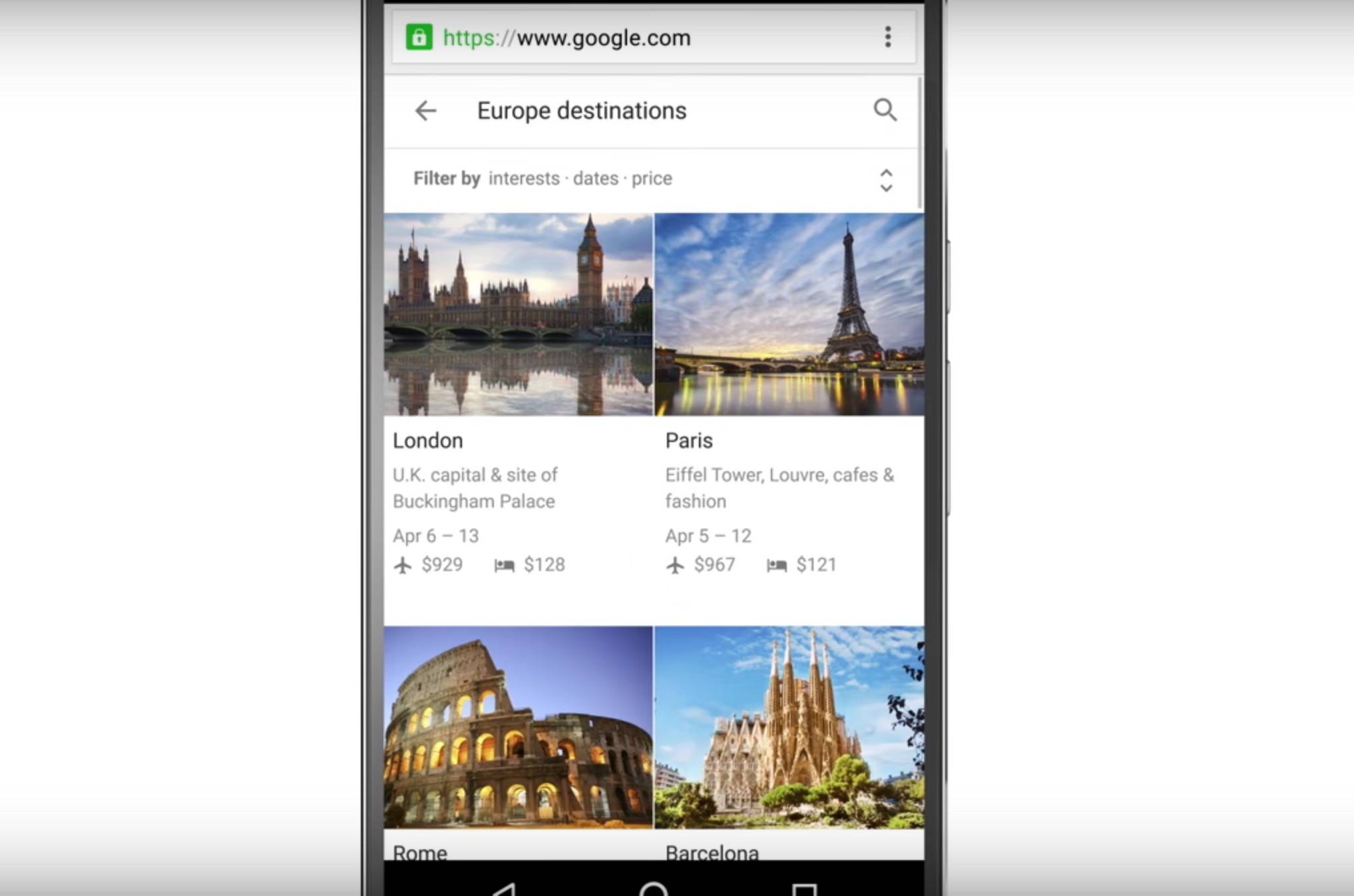In this unusual screenshot, the image is notably wide, yet the focus is on a smartphone with prominent drop shadows at both the top and bottom. The sides of the phone are visible, showcasing the sleek metal casing and reflective glass, although the top and bottom curves of the device are omitted. The bottom part of the screen, where the navigation bar starts, is partially cut off.

At the top of the screen, a green lock icon indicates a secure connection, followed by the URL in green "HTTPS://", which transitions into light gray, and the website "www.google.com" in black. Beneath the URL bar, within the search field next to the back button, the text "Europe destinations" is visible, along with options to "Filter by interest, dates, price."

The main content below this consists of four images representing different European destinations: London, Paris, Rome, and Barcelona. For London, there's a descriptive thumbnail showing Buckingham Palace with text overlay indicating "London, UK capital inside of Buckingham Palace, April 6th to 13th." Symbols for a plane and a bed display prices of $929 and $128 respectively, with a scenic view of the Thames and the iconic Clock Tower, including Big Ben, in the background.

To the right, Paris is depicted with a view from the Seine River highlighting the Eiffel Tower. The details state "Paris, Eiffel Tower, Louvre, cafes, and fashion, April 5th to the 12th." Flight and hotel prices are listed as $967 and $121 respectively. 

Rome is shown with the Colosseum, but the accompanying text is cut off. Similarly, the image of Barcelona features a renowned cathedral without any displayed information due to it being obscured by the navigational menu below.